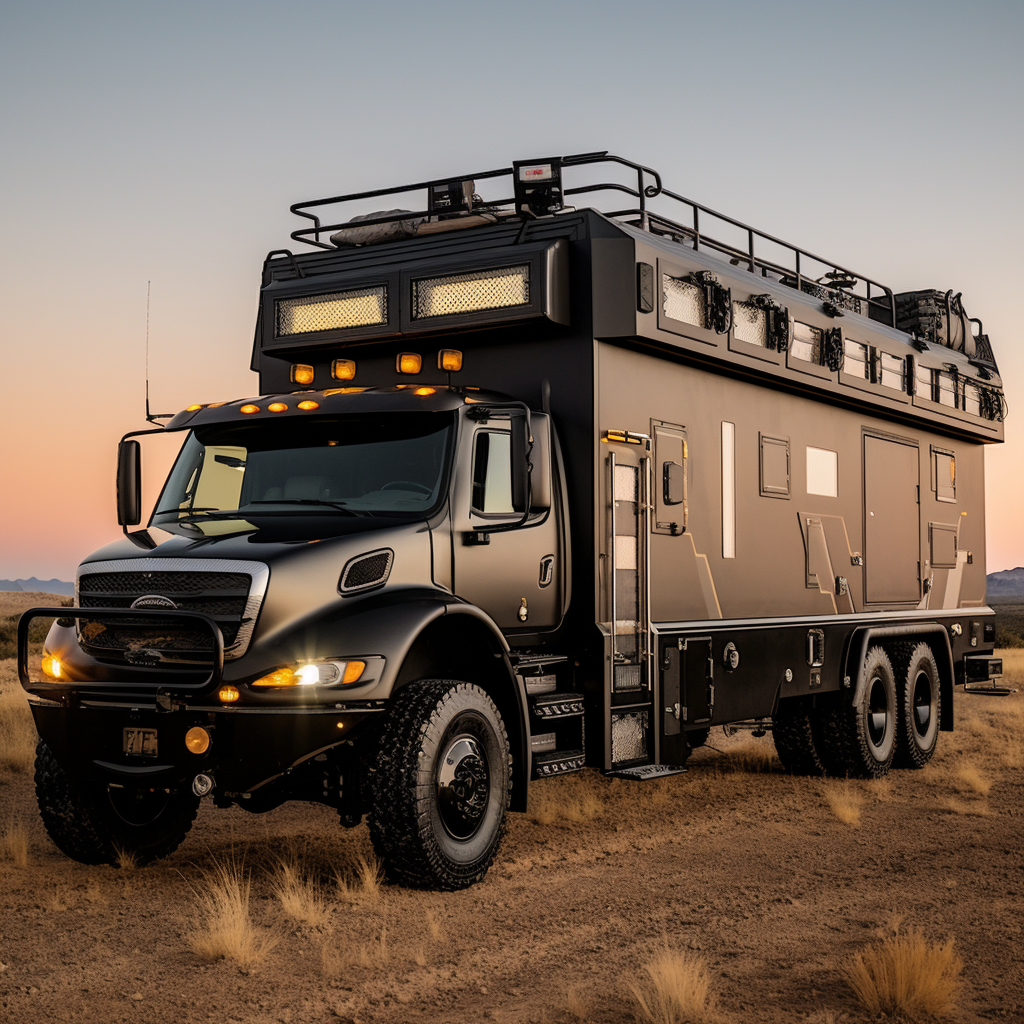This photograph captures a massive, militarized black truck resembling a fortified recreational vehicle, set against a stark desert backdrop. The vehicle's imposing front features a bullbar and has its headlights switched on, indicating an imminent dusk as a pink hue tinges the sky. Equipped with eight wheels in the rear and two in the front, the truck boasts a heavily armored, multi-functional rear section that could serve as both living quarters and secure transport. This rear compartment is punctuated by rows of small, metal-screened windows and includes doors on both sides, accessible via ladders and steps. Above, the roof is encircled by a railing system, possibly for storage crates or military personnel, adding to the vehicle's versatile yet enigmatic design. The scene is desolate, with only dirt and dry grass surrounding, emphasizing the truck's solitary presence. Despite no visible occupants, the battery drains as the truck's lights remain on, casting an ominous glow over the deserted terrain.